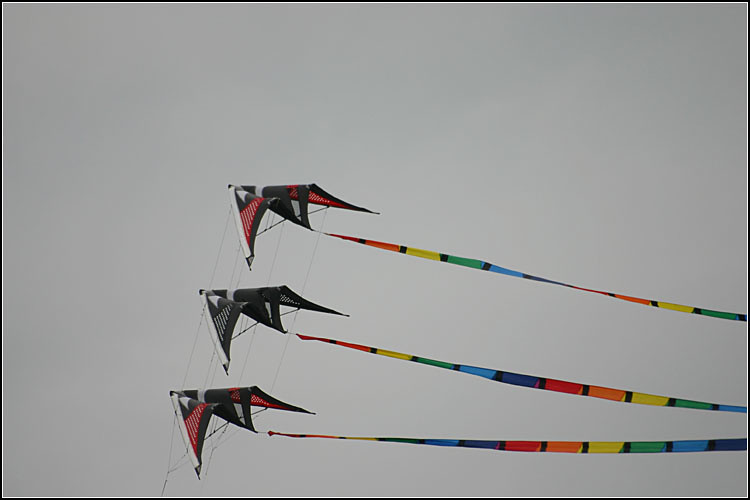This photograph showcases a trio of paper airplane-shaped kites soaring against a backdrop of a very gray, overcast sky. The kites, arranged in a triangular formation, possess striking color patterns: each has a black middle section, while the top and bottom kites feature red wings and the middle kite sports black wings. Tethered together by thin black strings, these kites create an illusion of a unified structure. Trailing behind each kite are long, vibrant tails comprised of repeating rainbow sequences—red, orange, yellow, green, blue, and purple—adding splashes of color to the otherwise monochromatic sky. The strings and tails extend off the right edge of the photograph, implying a continuous motion beyond the frame.